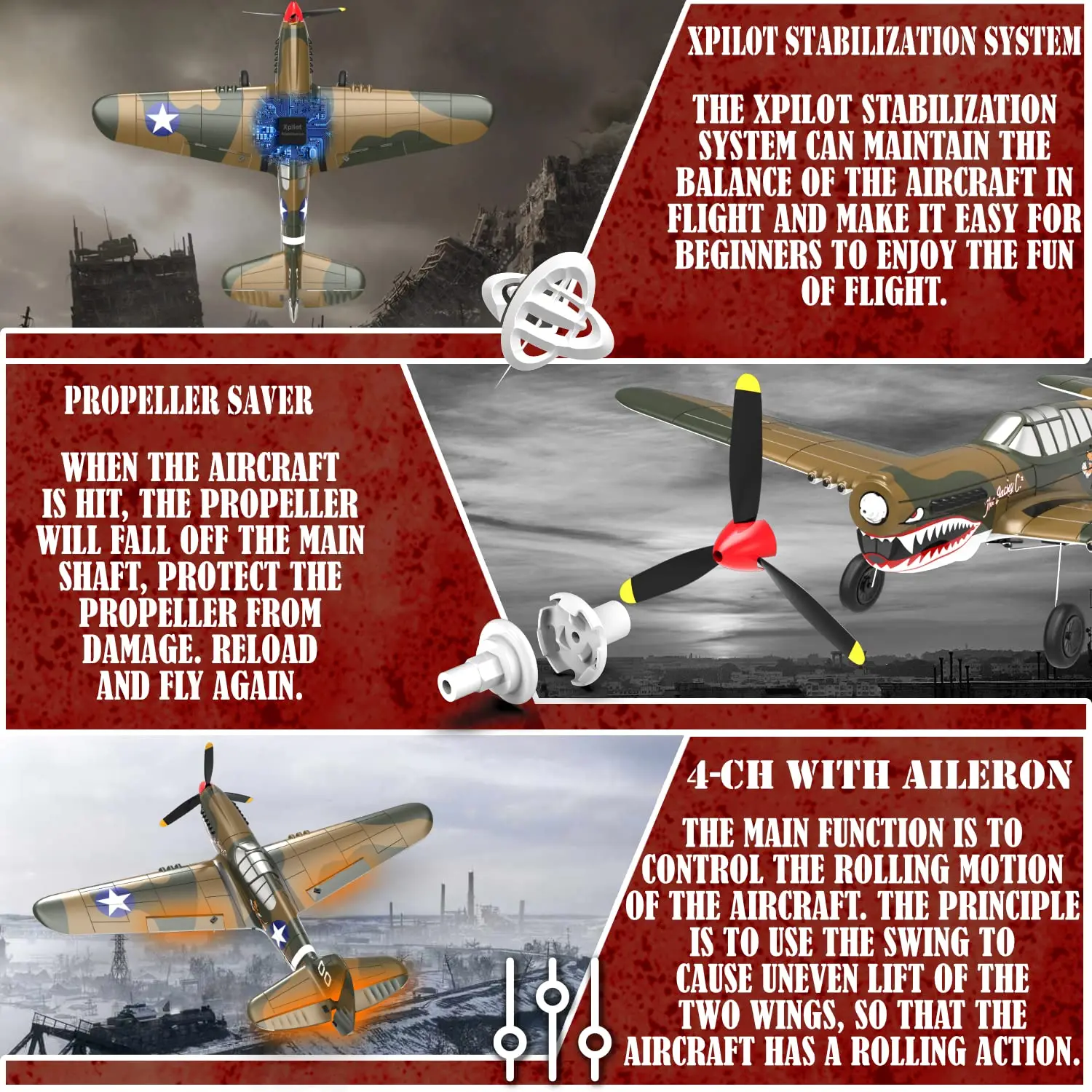The image showcases three vintage-style model airplanes, each section detailing different features and parts of the planes. The first section, featuring a U.S. camouflage-colored airplane with a white star, highlights the "X-Pilot Stabilization System," which helps maintain the aircraft's balance during flight, making it suitable for beginners. The second section emphasizes the "Propeller Saver," explaining that the propeller, depicted in red with black blades and yellow tips, will detach upon impact to prevent damage and can be reloaded for continued use. The final section describes the "4CH with Aileron" system, which controls the airplane's rolling motion by causing uneven lift between the wings. The aircraft in this section also bears a white star and appears against a backdrop resembling a bombed-out city, suggesting a World War II theme. The text throughout the image is white, capitalized, and set against red backgrounds, indicating it could be from advertising or packaging for these model airplanes.